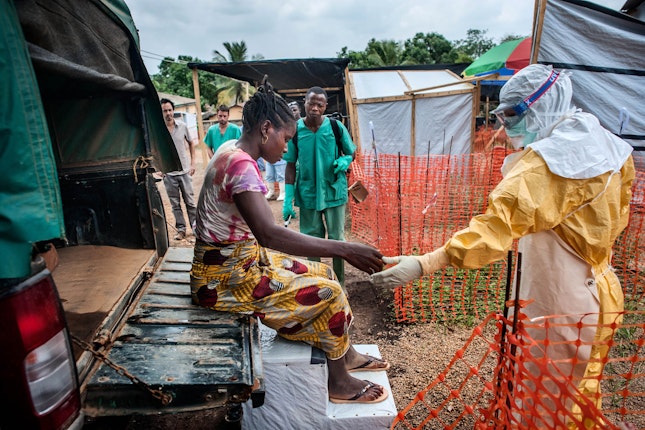This photograph captures a scene in an outdoor refugee camp, characterized by temporary orange safety netting used as fences. In the foreground, a young black woman with her hair up and wearing hoop earrings, a pink and purple tie-dye shirt, a long skirt with a red fruit pattern, and sandals is seated on the bed of a truck. She appears to be in the process of being helped down by an individual in full protective gear, which includes a yellow paper suit, latex gloves, goggles, and a white paper hood. This person's gloved hands are reaching out to assist the woman, whose gaze is directed downward as she accepts the help.

To the right, a black man dressed in green scrubs and matching green gloves stands nearby, observing the situation. In the background, makeshift shelters built from wooden planks and tarps are visible, with additional figures present – one person also in green scrubs and another dressed in a tan polo shirt and dark pants. The setting is framed by green trees, some resembling palm trees, set against a gray, cloudy sky. The overall atmosphere conveys the urgency and provisional nature of the camp.